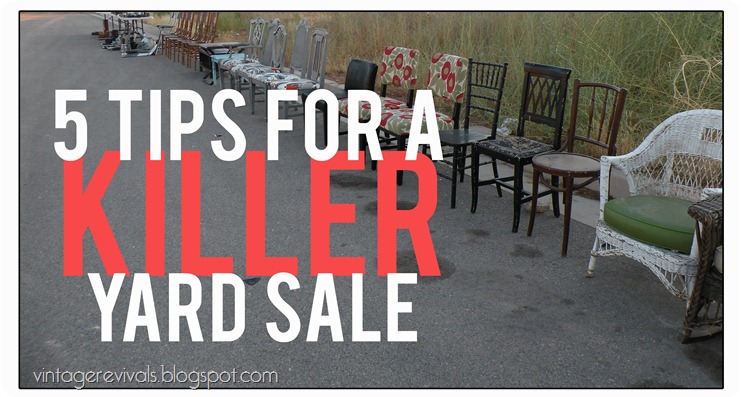The image is a visually striking advertisement in landscape mode, promoting a blog article on yard sale tips, as indicated by the text overlay. The central text, "5 Tips for a Killer Yard Sale," is prominently displayed, with "killer" in bold red letters and the rest in white. In the bottom left corner, the URL "vintagerevivals.blogspot.com" is clearly visible. The photograph features approximately 20-25 assorted chairs lined up along a paved roadside with some oil spots, set against a backdrop of tall, green grass interspersed with patches of brown. The chairs vary in style and condition, including a notable white wicker chair with a green cushion, several wooden chairs in walnut and dark wood finishes, and cushioned chairs with red floral and green leaf patterns. This eclectic collection of second-hand furniture vividly illustrates the essence of a dynamic yard sale.